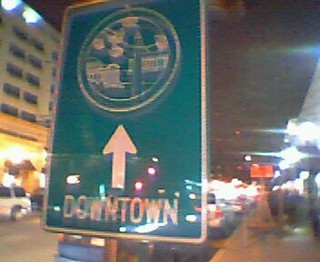The image shows a low-resolution, nighttime photograph of a reflective street sign situated on a city sidewalk. The rectangular sign is a greenish-blue or teal color with white text, featuring the word "DOWNTOWN" in all capitals near the bottom and a thick white arrow pointing upward. Above the arrow, within a two-layered circular shape, there appears to be an unclear drawing, possibly of a building or group of buildings. Surrounding the sign, the nighttime city street is visible, with a light tan or white building with dark windows on the left, which could be a tall structure like a hospital or office. The right side of the image shows a gray sidewalk in front of stores and buildings, with some people and blurred lights creating streaks. Cars are parked along the sides of the street, and there are additional red signs and various lights scattered throughout the background, contributing to the urban atmosphere. The photo quality suggests it may have been taken with an older personal camera or camcorder, resulting in the grainy and blurred details.